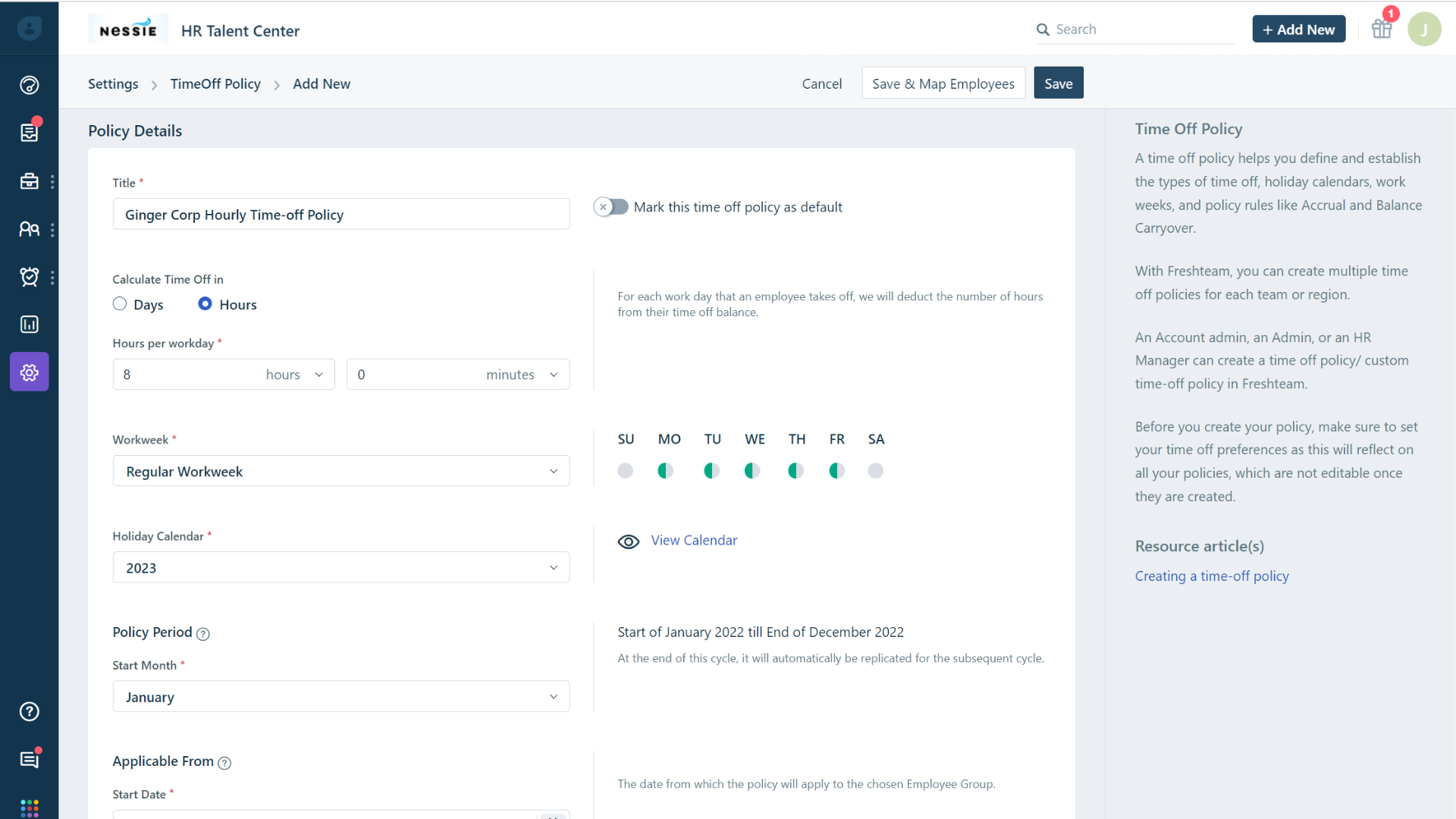**Screenshot Overview of HR Talent Center Utility Page**

The image is a screenshot of a utility page from a web application. In the upper left corner, there is a company logo displaying "NESSIE" in black capital letters. Above the letter "I" in the logo, there is a small blue icon resembling a bird in a tilted line shape. 

To the right of the logo, the header "HR Talent Center" is prominently displayed in capital letters. 

A thin, dark blue sidebar runs down the left side of the page, featuring various white icons. The main section of the page includes a light gray menu bar at the top with options labeled "Settings," "Time Off Policy," and "Add New." 

Beneath the menu, a slightly darker gray section titled "Policy Details" is present. This section contains a square display area. At the top of this area, the title reads "Ginger Corp Hourly Time Off Policy." Below this title, there is an option to "Calculate time off in" with choices between days or hours. 

On the right side of the page, another sidebar provides a detailed explanation of the time off policy. It begins with a header titled "Time Off Policy" and continues with a description stating that a time off policy helps define and establish various types of time off, holiday calendars, work weeks, and policy rules such as accrual and balance carryover, among other details. 

This screenshot captures an interface designed to assist users in configuring time off policies efficiently.